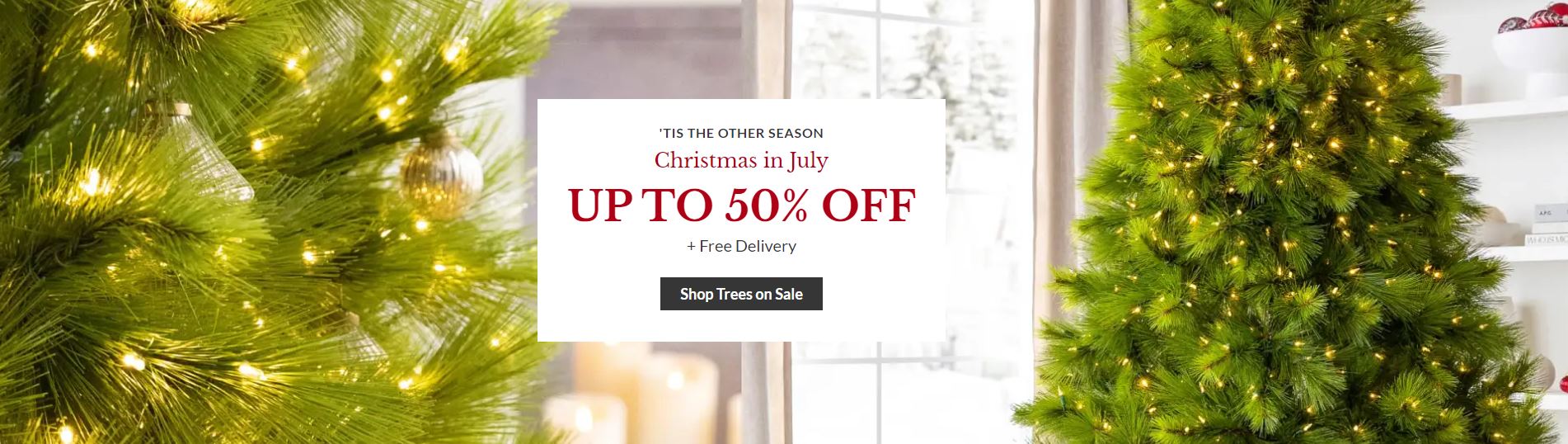The advertisement features a festive rectangular design that is approximately three times wider than it is tall. On the left third of the image, there is a close-up shot of a Christmas tree, showcasing its vibrant green branches adorned with yellow lights and a single silver ornament hanging to the right. The background consists of a subtle grey wall transitioning into a darker grey halfway through the image.

Near the center, a window with bright, almost blown-out light filters through a slightly visible brown curtain. Adjacent to the window is another lush green Christmas tree, festooned with yellow lights, extending from just below the top to just above the bottom of the frame.

To the right of this tree, a white wall houses a set of shelves. The top shelf holds a white bowl filled with red items, the middle shelf features a row of books that partially extend beyond the edge, and the bottom shelf displays an arrangement of round objects in brown and red hues.

Centrally placed, overlapping the window and extending towards the right-side wall, is a prominent white square. At the top, it reads “‘Tis the other season” in small black font. Below, in bold red letters, it announces “Christmas in July” with “Up to 50% off” highlighted in large red text. Beneath this, smaller black font states “plus free delivery.” A black tab at the bottom contains white text that encourages viewers to “Shop Trees on Sale.”

This ad effectively combines holiday cheer with enticing offers, drawing attention to the seasonal sale.